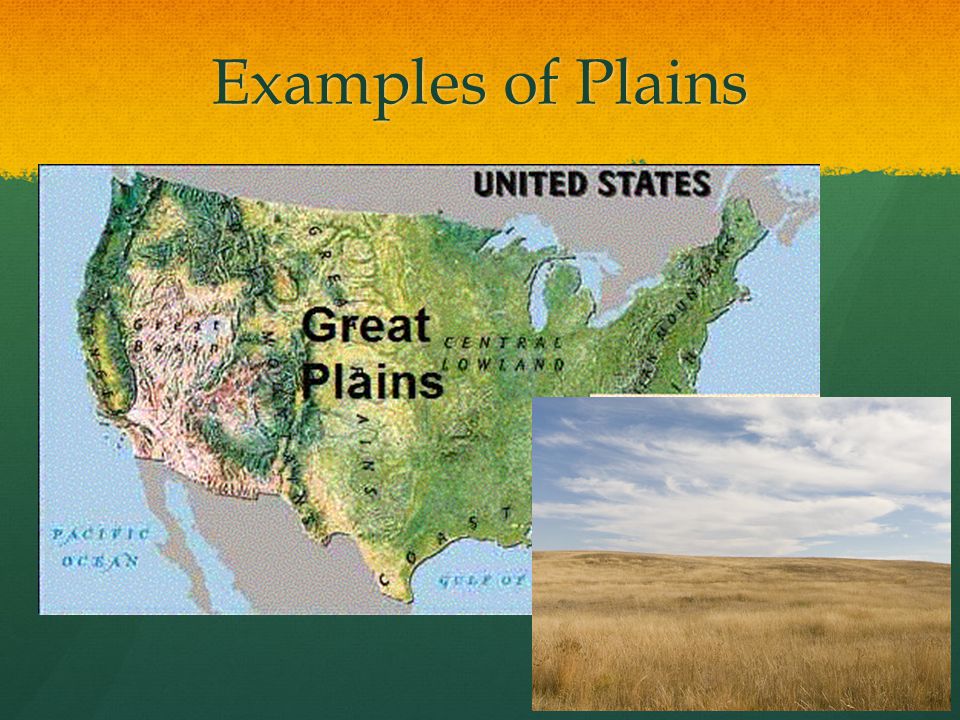The image is a detailed map of the United States, primarily showcasing various types of plains within the country. The map is divided into multiple sections that depict different geographic features. The top of the map features the text “Examples of Plains” on an orange-colored background. The central part of the map prominently displays the “Great Plains” in bold print. Adjacent to this, towards the right, the “Central Lowland” is labeled. The map itself is colored to indicate different landforms: green for plains and brown for mountainous regions. On the left side of the map, the text “Pacific Ocean” is visible, while on the lower right, it reads “Gulf of” and “Coast” around the Texas area. Additionally, there is an inset image in the lower right corner showing a field of tall, golden-brown grass under a blue sky scattered with white clouds, representing a typical plains landscape. This inset provides a visual example of the plains described on the map.